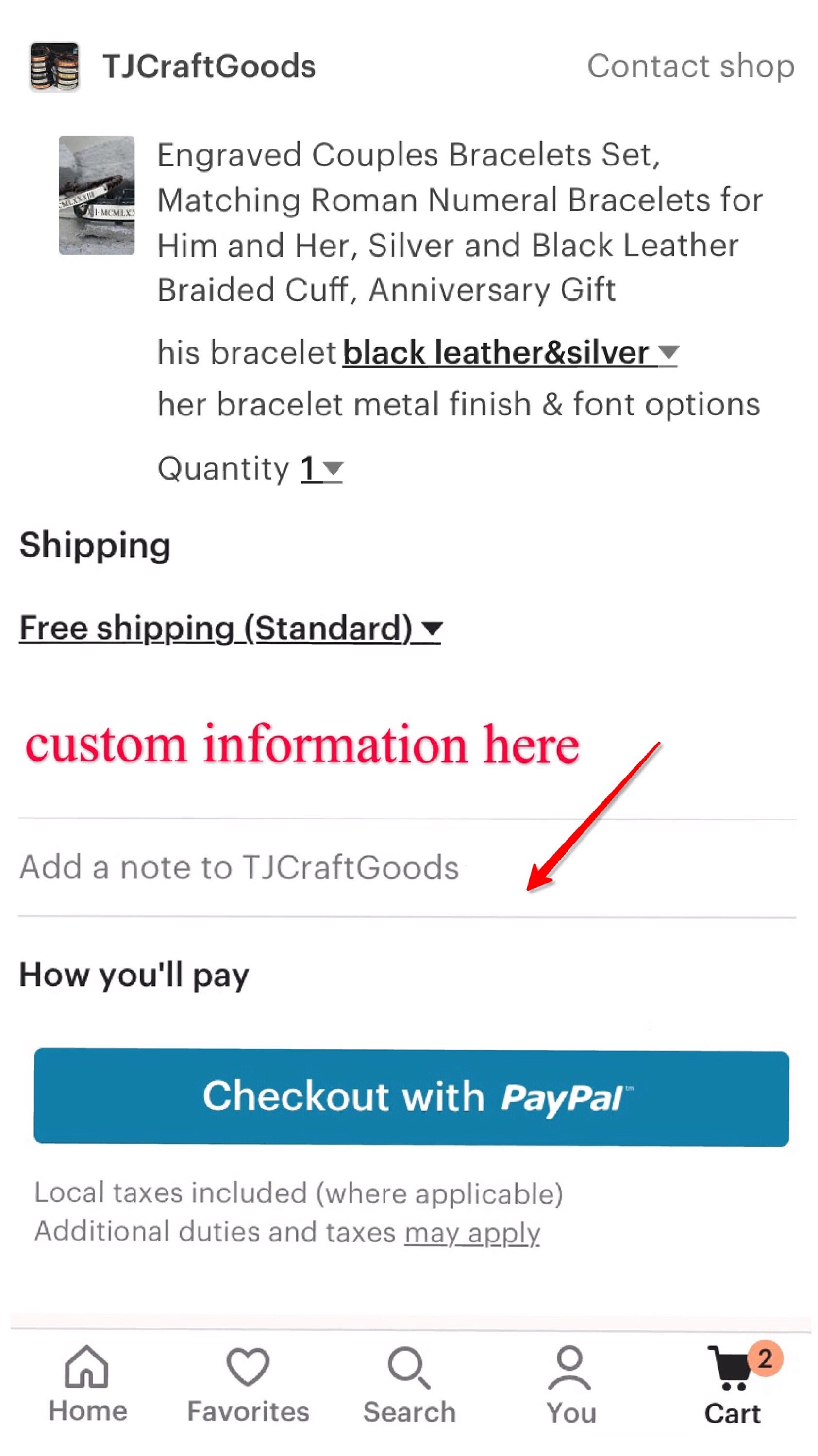The image depicts a product page for TJ Craft Goods, an online shop specializing in personalized items. At the top left, the shop name, "TJ Craft Goods," is prominently displayed, while to the right, a "Contact Shop" option is available. Central to the image is a detailed description of an item titled "Engraved Couples Bracelet Set." The set includes matching Roman numeral bracelets for couples, featuring a black leather and silver bracelet for him, and a silver metal bracelet for her, with customizable font options.

Below the item description is a quantity selector, currently set to one. The shipping section indicates "Free Shipping" with the default set to "Standard." A red-highlighted section labeled "Custom Information Here" invites customers to provide specific customization details. Directly beneath this, an option to "Add a Note to TJ Craft Goods" is marked with a red arrow pointing towards it for easy navigation.

Further down, information on payment options is provided under "How You'll Pay," with a notable blue button labeled "Check Out with PayPal." Additional financial details mention that local taxes are included where applicable, with a caveat that extra duties and taxes may apply.

At the bottom of the screen, navigation buttons are displayed: "Home," "Favorites," "Search," "You," and a "Cart" button indicating that there are currently two items in the customer's cart. This comprehensive page layout facilitates a seamless shopping experience for users looking to purchase from TJ Craft Goods.